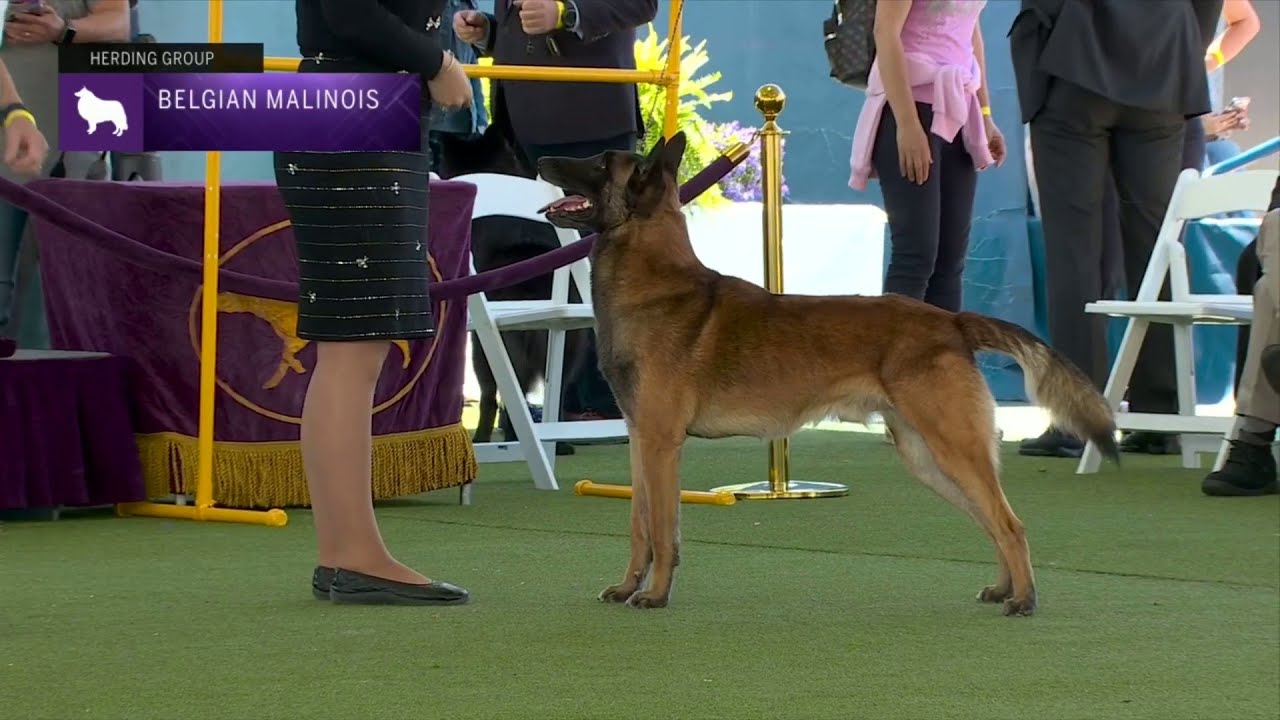The image captures a lively scene at a dog show focused on a Belgian Malinois and its handler, who is a woman in a dark blue skirt and flats. The dog stands attentively, awaiting a command. It has a tan coat with striking black accents on its face and tail, resembling a smaller German Shepherd. In the backdrop, a green outdoor carpet covers the central arena where judges are seated and observers are gathered. Prominently, a table with a purple satin cloth and golden fringe displays a silhouette of a dog and the words "Belgian Malinois." Visible attendees include a man in a suit, a girl with a lavender sweatshirt tied around her waist, and white chairs. A label in the upper left corner of the image reads "Herding Group," emphasizing the breed's association. The scene hints at the poised anticipation and rigorous training that characterize such events, showcasing the athleticism and obedience of these intelligent canines.